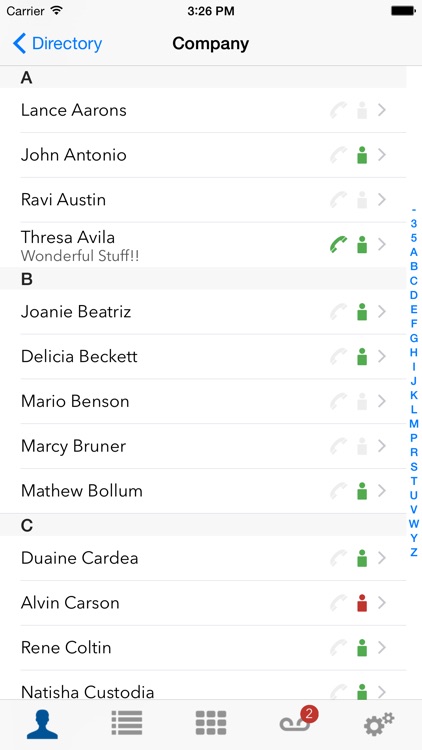Screenshot of a mobile device displaying a contact directory. At the top, the screen indicates it is 3:26 p.m., with the mobile carrier and Wi-Fi signal visible, and the device shows a fully charged battery. The directory is titled in blue font, with "Company" listed in black. Names listed include Lance Aarons, John Antonio (who has a green profile icon and phone symbol), Robbie Austin, Teresa Avila, Joni Beatriz, Delicia Beckett, Mario Benson, Marcy Bruner, Matthew Bullum, Duane Cardia, Alvin Carson (with a red icon), Renee Colton, and Leticia Custodia. Most contacts feature green profile icons indicating availability, with the exception of Alvin Carson who has a red icon.